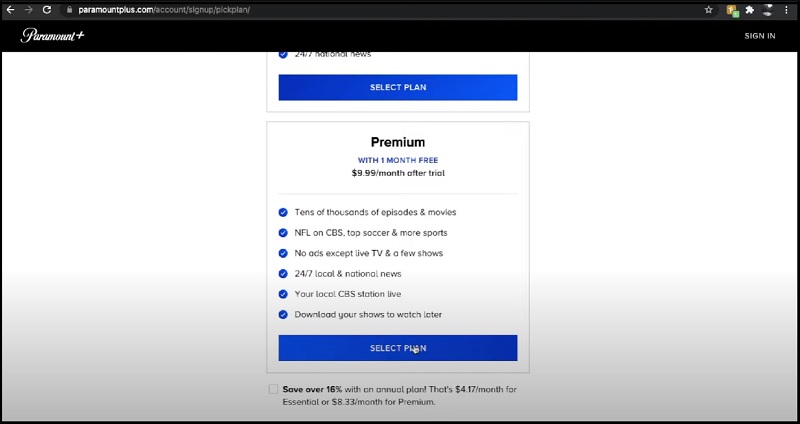The image displays a webpage on the Paramount Plus website at the URL paramountplus.com/account/sign-up/pick-play. The toolbar contains several icons: a star, two unidentified icons (one yellow and one green), another white icon, two more unidentified icons, and a three-dot menu on the far right. Below this toolbar, the Paramount Plus logo is prominently displayed, with the "Sign In" option positioned to the far right.

The main content area features a white screen overlayed by a subscription plan selection box with a prominent blue button labeled "Select Plan." The highlighted plan reads "Premium" and offers a one-month free trial followed by a $9.99 per month subscription fee. Features of the Premium plan are listed with blue and white check marks, including:

- Tens of thousands of episodes and movies
- NFL on CBS, top soccer, and more sports
- No ads except for live TV and a few shows
- 24/7 local and national news
- Live streaming of your local CBS station
- Download options for shows to watch later

The cursor in the image is positioned over the "Select Plan" button, indicating the user is about to choose this plan. An additional box highlights the option to save over 16% with an annual plan, breaking down the monthly cost to $4.17 for the Essential plan or $8.33 for the Premium plan.